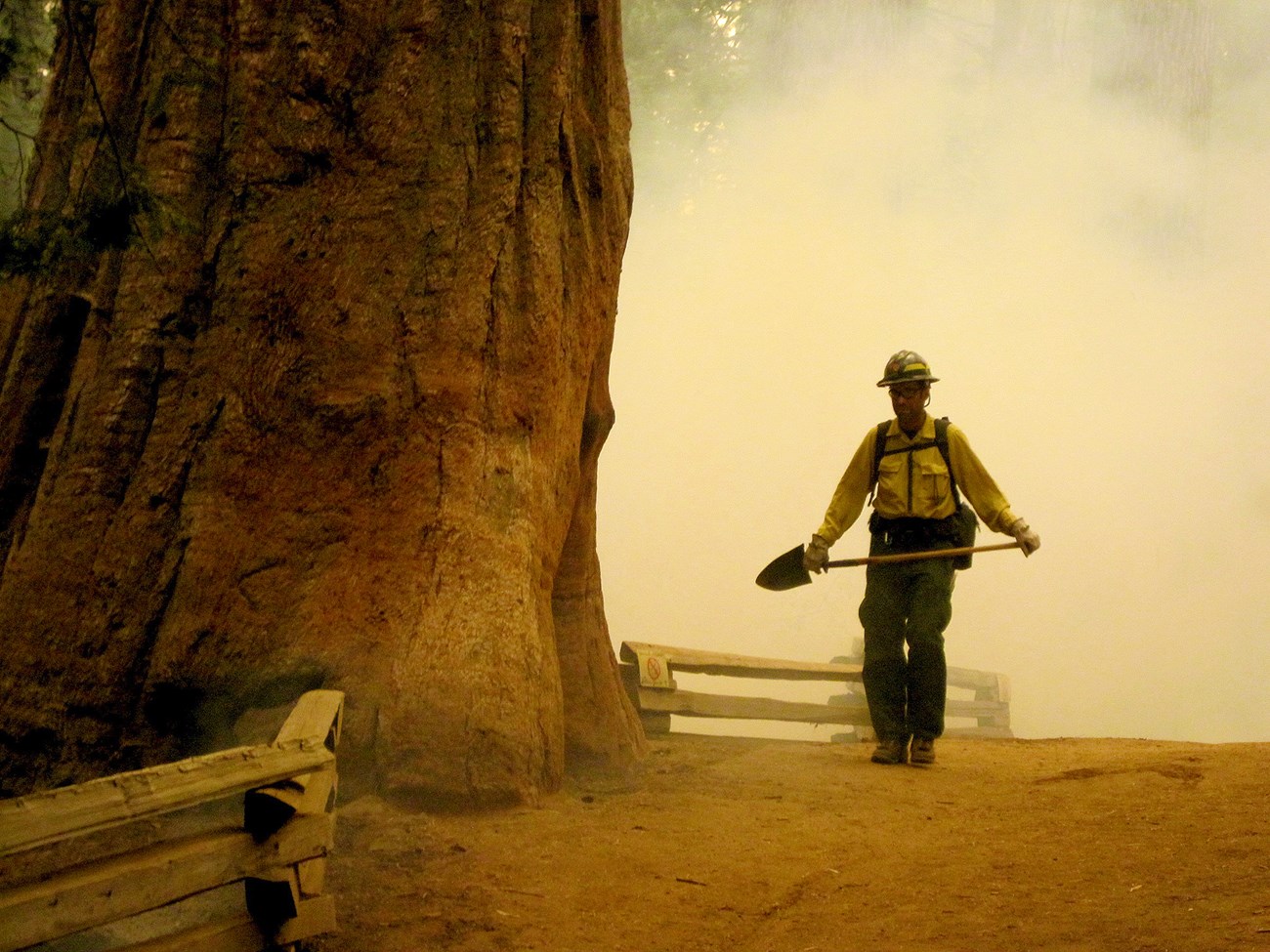The photograph captures a man standing in a dense forest, likely in Northern California, next to a towering and thick redwood tree with a textured bark in various shades of brown, tan, and red. The massive tree dwarfs the man, who is dressed in a yellow long-sleeved work shirt, dark green work pants, sturdy boots, and a silver helmet equipped with a light, resembling a miner’s or firefighter's gear. He holds a shovel with both hands, its blade facing downward, as small wooden fences dot the dirt and sandy ground around him. The scene is enveloped in a haze of white smoke or fog, adding an element of mystery and suggesting the possibility of nearby mining activity or a fire. The overall setting emphasizes the interaction between man and the majestic, natural environment.